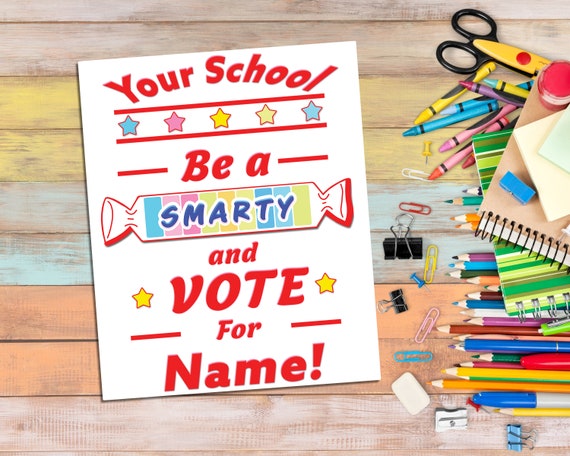The image is a vibrant and detailed graphic, presumably created for a school campaign, possibly for student council elections. Set against a background that looks like a painted wooden table, featuring light hues of yellow, blue, and red, the main section of the graphic is a white template. At the top, in bold red text, it reads "YOUR SCHOOL." Below it, the phrase "BE A SMARTY" appears, where "SMARTY" is designed to mimic the logo of Smarties candy and is spelled out in blue. The text continues with "AND VOTE FOR" followed by a placeholder for a candidate's name. Along the right-hand side of the poster, there's a selection of colorful school supplies such as pencils, crayons, colored pencils, scissors, notebook, erasers, paperclips, pushpins, a pencil sharpener, and a spiral notebook. All these elements together make the graphic both eye-catching and functional, emphasizing school spirit and the election theme.